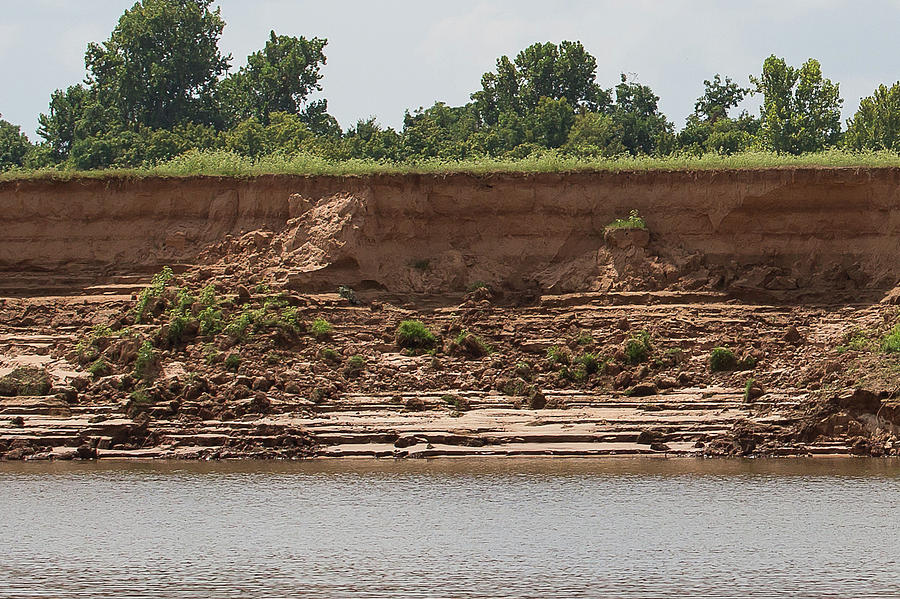This photograph captures a natural outdoor scene with a bright, sunlit ambiance against a gray sky. The landscape features a body of murky, brownish water set before a steep, angular cliff of clay-brown and reddish dirt, suggesting it was artificially excavated. Above the cliff, lush green fields and numerous trees line the horizon, while the cliff face itself is rigid, rocky, and layered, dotted with small green shrubs. In front of this dugout land, a variety of green plants and small shrubs thrive, adding to the vibrant, yet rugged beauty of the scene.